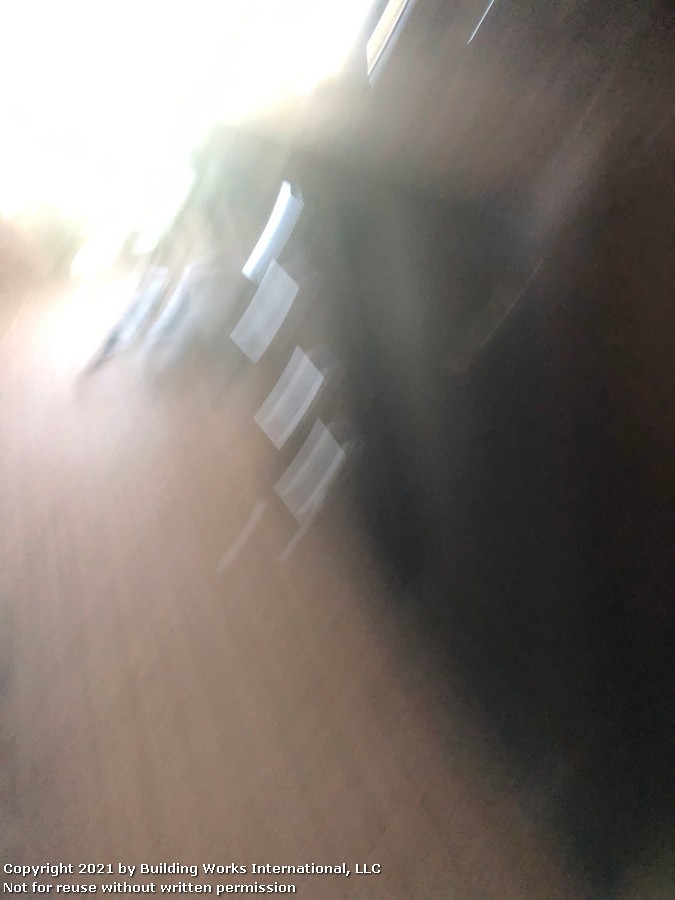The image is an extremely blurry and out-of-focus photograph, making specific details difficult to discern. In the top left corner, there is a glaring white overexposed area, likely a window with sunlight streaming through. To the left, a vertical strip in brown hinting at floorboards or a counter stretches from top to bottom. On the right side, dark and tan indistinguishable shapes dominate the scene, while closer to the center, a series of four silvery grey squares or box-like shapes can be vaguely seen. Spread across the bottom left corner, amidst a brownish background that might resemble a floor, is a clear textual overlay in white letters that reads: "Copyright 2021 by Building Works International LLC, not for reuse without written permission." The image appears to capture a moment with significant motion blur, possibly from a camera phone in shakiness, adding to the overall indiscernible nature of the photograph.